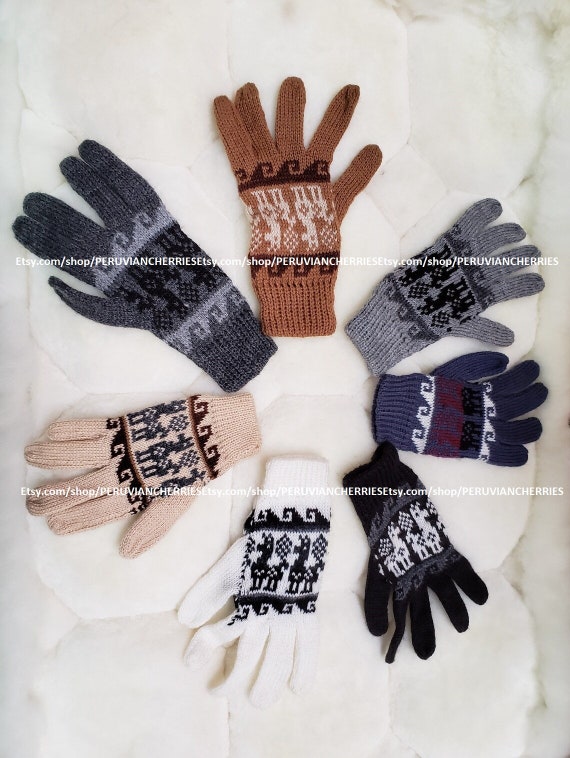This image showcases an appealing selection of handmade gloves arranged in a circular formation, reminiscent of the numbers on a clock. These gloves are displayed on a pristine white quilted background. Starting from the 12 o'clock position, the gloves are colored brown, light gray, blue, black, white, tan, and dark gray, forming a charming palette.

Each pair of gloves features a delightful llama pattern, with llamas placed upside-down so they face the fingers of the gloves. The brown gloves feature a black border adorned with white llamas. The light gray gloves have a dark gray border with black llamas. The blue gloves sport a white border with distinctive red-topped black-bottomed llamas. Black gloves are complemented by a gray border with white llamas, while the white gloves have a black border featuring black llamas, as do the tan gloves. Lastly, the dark gray gloves showcase a light gray border with black llamas.

A watermark stretches across the image, appearing about one-third and two-thirds down from the top, reading "etsy.com/shop/peruviancherries," and it's repeated throughout the picture.